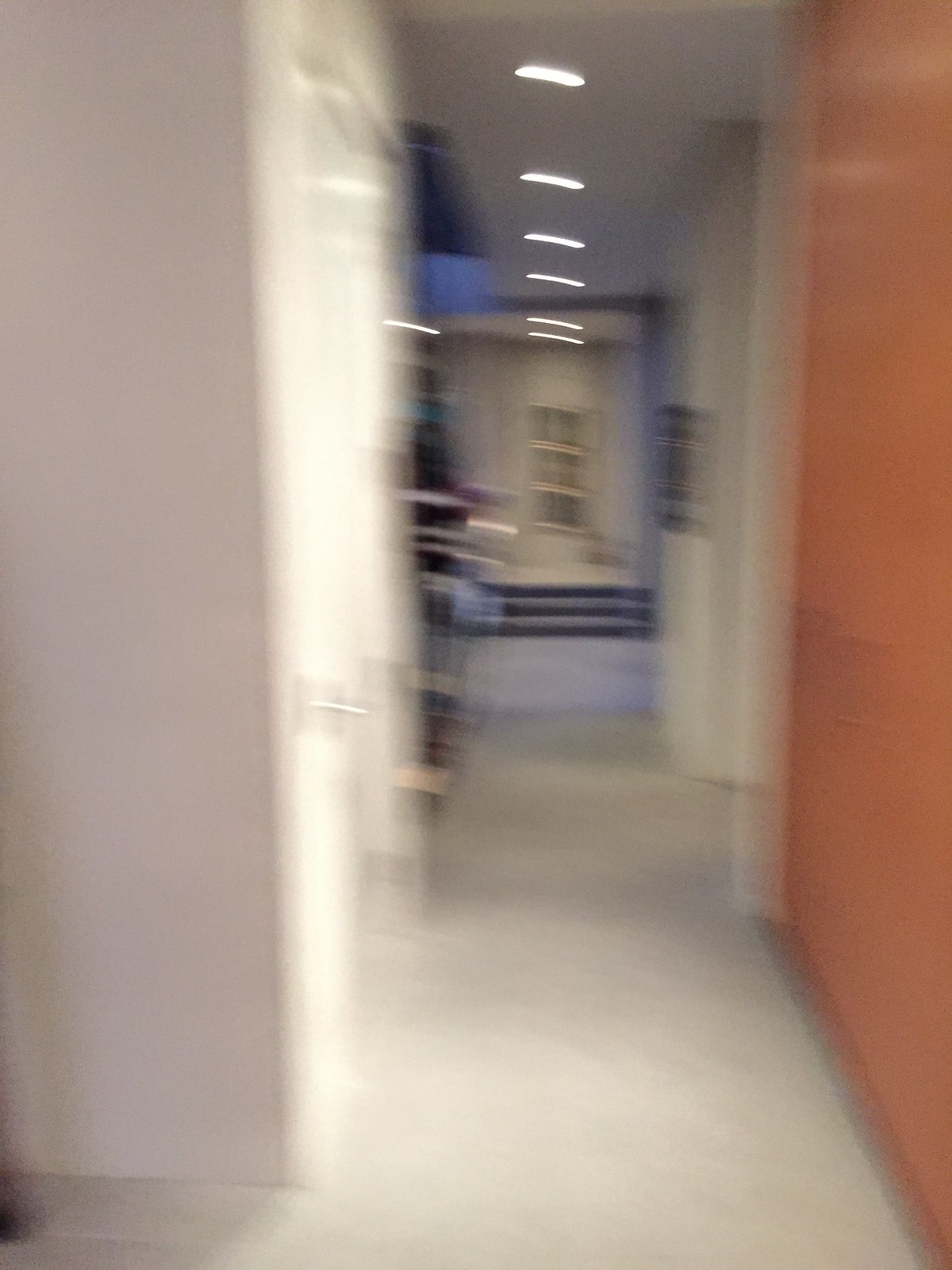This extremely blurry photograph captures an interior hallway of a residence, viewed straight down its length. The right wall is a coral or darker orange color, reflecting light from evenly spaced, round ceiling lights. The left wall is white, and there seems to be a turn or corner to the left. The floor is light-colored, possibly gray tile or white carpeting. At the end of the hallway, there are three horizontal black lines that may indicate steps. Above these steps, the wall continues in white, framing a window or door with a decorative glass panel, which is divided into multiple squares and has a dark gray background. The perspective suggests the camera was moving, adding to the image's blurriness. There is also an open doorway along the hallway and possible greenery visible in the distance through the opening to the left.